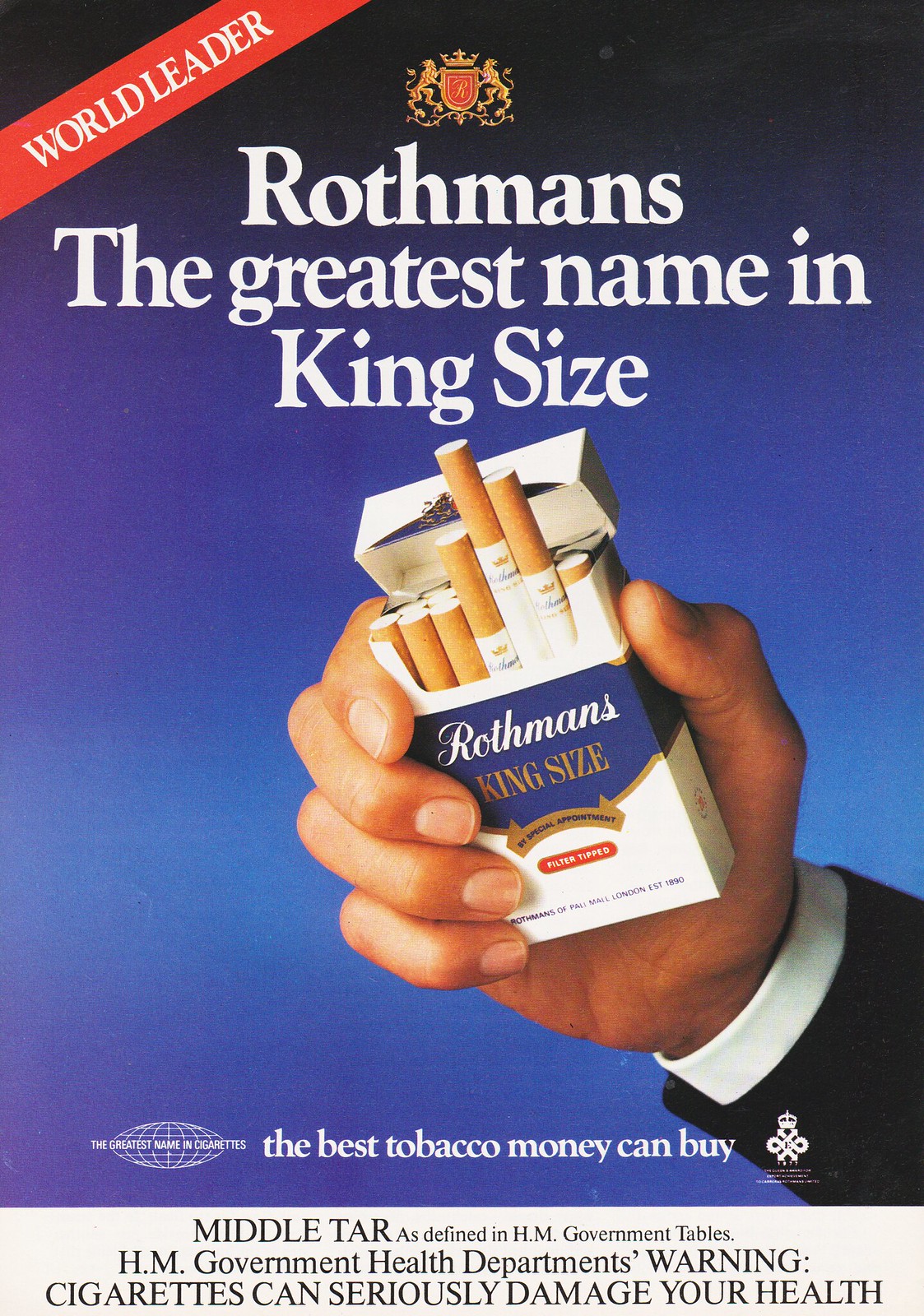This image is an advertisement for Rothman's King Size Cigarettes, possibly from a magazine. The central focus is a male hand, dressed in a white shirt and black coat, holding an open pack of Rothman King Size Cigarettes, with some cigarettes protruding from the pack. The pack is a striking white and blue with gold lettering. The background features a gradient of blue shades, transitioning from almost black at the top to a lighter blue and then back to dark blue. 

In the top left corner, there's a diagonal red banner with white lettering reading "WORLD LEADER." Across the top of the advertisement, in white letters, it says "Rothman's, the greatest name in king size." Below the image of the hand and cigarette pack, in white text, it reads "the best tobacco money can buy," flanked by logos on each side. 

At the bottom of the advertisement, a gray bar contains a health warning in black lettering, mandated by the HM Government Health Department, stating, "Cigarettes can dangerously damage your health."